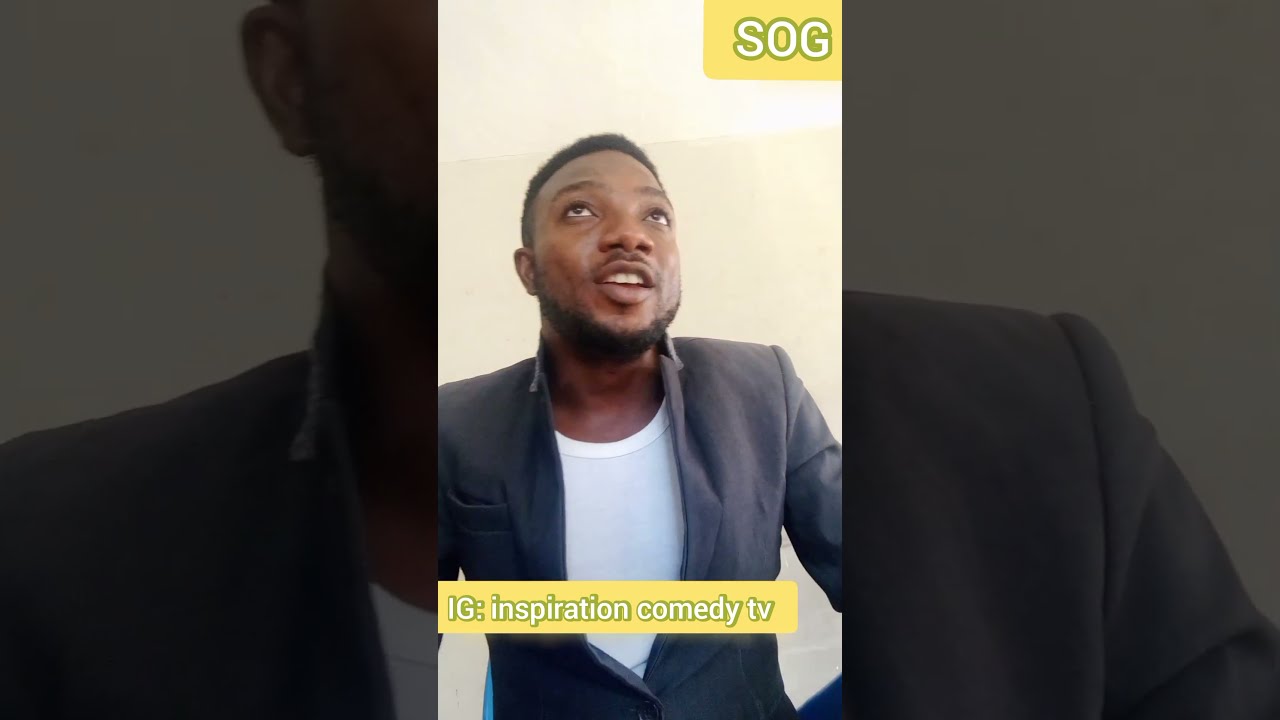The image features an African-American man with short, slightly longer hair on top, and a well-groomed black beard and mustache. He is dressed in a dark gray or black suit jacket over a white t-shirt. The man, who is the focal point of the image, stands centered, with his arms resting by his sides and a smile directed upwards, possibly towards the sky. The background is subtle cream or white, maintaining a neutral tone. In the top right corner, there is a yellow box containing the letters "S-O-G" in white with a green outline. Similarly, near the man's chest level, another yellow box displays the text "IG: Inspiration Comedy TV" in white with a green outline. The image appears to be a snapshot, potentially from a comedy clip or performance, given the inscriptions. It captures the man from about the waist up, emphasizing his composed and approachable demeanor.